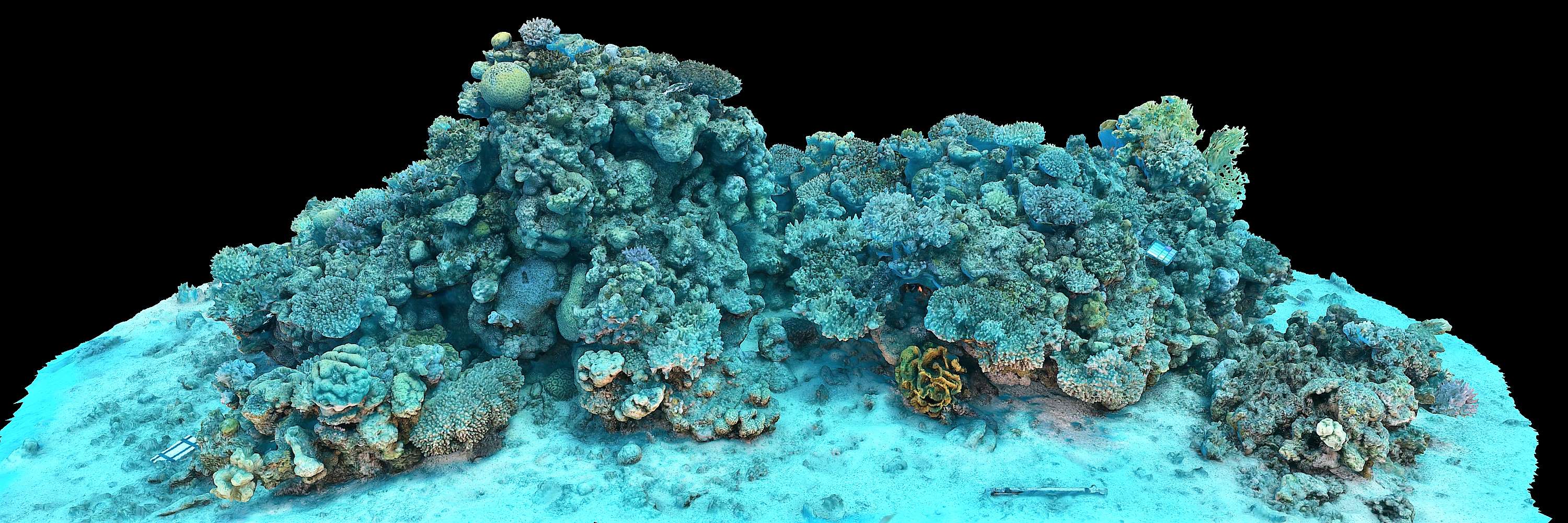This is a detailed 3D render of a coral reef resting on a light blue seafloor, with a stark black backdrop that gives the image a cut-out appearance. The rectangular, horizontally oriented image showcases the intricacies of the reef with various shades of blue and gray, alongside hints of green and yellow, particularly towards the bottom center. The reef features outcroppings, shells, and rocks, adding to its realistic and textured look. Notably, there is an area on the left where the render seems to have failed, revealing a white and blue striped patch. Additionally, a mysterious bar-like object is situated in the sand near the bottom right. This 3D imaging photo, likely generated by AI to monitor and potentially aid in conserving coral reefs, aims to provide a high-resolution map of underwater ecosystems.